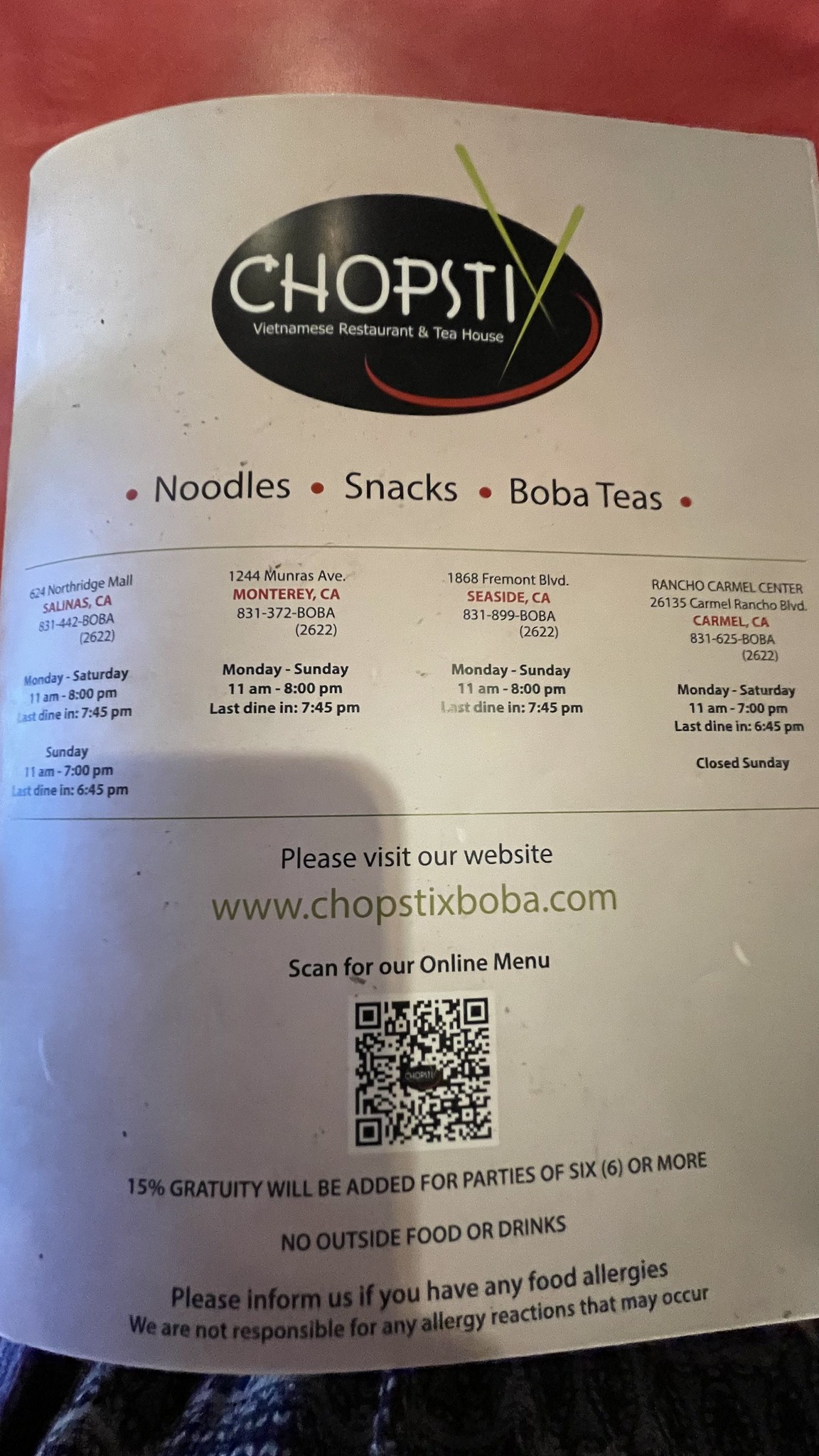This photograph showcases the menu of a dining establishment named "Chopsticks." At the top of the menu sits the restaurant's logo, enclosed within a black oval. The word "Chopsticks" is prominently displayed in white lettering, with the unique detail of the "X" being formed by two green chopsticks intersecting each other. A red crescent accentuates the logo, underlining the name.

Beneath the logo, their website "www.chopsticksboba.com" is listed, along with a QR code that offers a convenient way to access the online menu. Highlighting the restaurant's specialties, the text "Noodles, Snacks, Boba Teas" is positioned prominently below the website information.

Further down, the menu provides the addresses of their various locations, all of which are based in California. Notable locations include Seaside, Carmel, and Monterey. Due to a curvature in the menu, the fourth location is not entirely visible.

At the bottom of the menu, there are additional notes for customers: a 15% gratuity will be added for parties of six or more, no outside food or drinks are permitted, and patrons are requested to inform the staff of any food allergies.